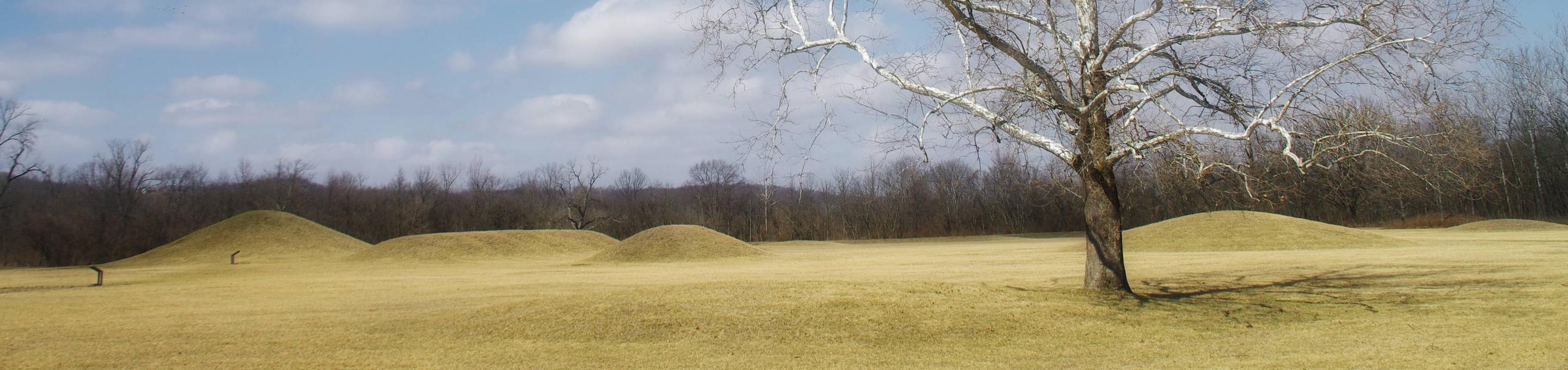The panoramic outdoor image captures a bright, sunny day with a vivid blue sky adorned with scattered clouds, some fluffy white and others tinged with light gray. The landscape features a flat expanse punctuated by small, peculiar mounds—three with pointed tops and one with a flat top—suggesting possible historic significance, perhaps Native American mounds accompanied by historic markers for visitors to read about them. A solitary, large tree dominates the foreground, its bare, white-branched silhouette casting a stark shadow on the ground to the right. The rest of the image is populated by a scattered row of thin, brown trees, also devoid of leaves, indicating the season is likely fall as the grass below fades from green to a dull yellow. In the very distant background, faint silhouettes of mountains add depth to this simple yet evocative scene.